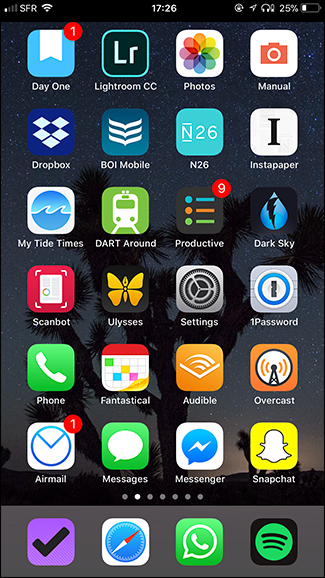Screenshot of an iPhone home screen displaying a variety of apps. The iPhone in question unusually does not resemble a typical iPhone interface at the top. The screen includes apps such as Day One, Lightroom CC, Photos, Manual, Dropbox, Boy Mobile, N26, Instapaper, Mai Tai, Times, Dart Around, Productive, Dark Sky, Scanbot, Ulysses, Settings, 1Password, Phone, Fantastical, Audible, Overcast, Airmail, Messages, Messenger, Snapchat, Spotify, WhatsApp, Safari, and an unidentified app with a checkmark icon. The status bar shows only one bar of cellular signal but full Wi-Fi signal. The battery is at 25%, and the time displayed is 17:26.